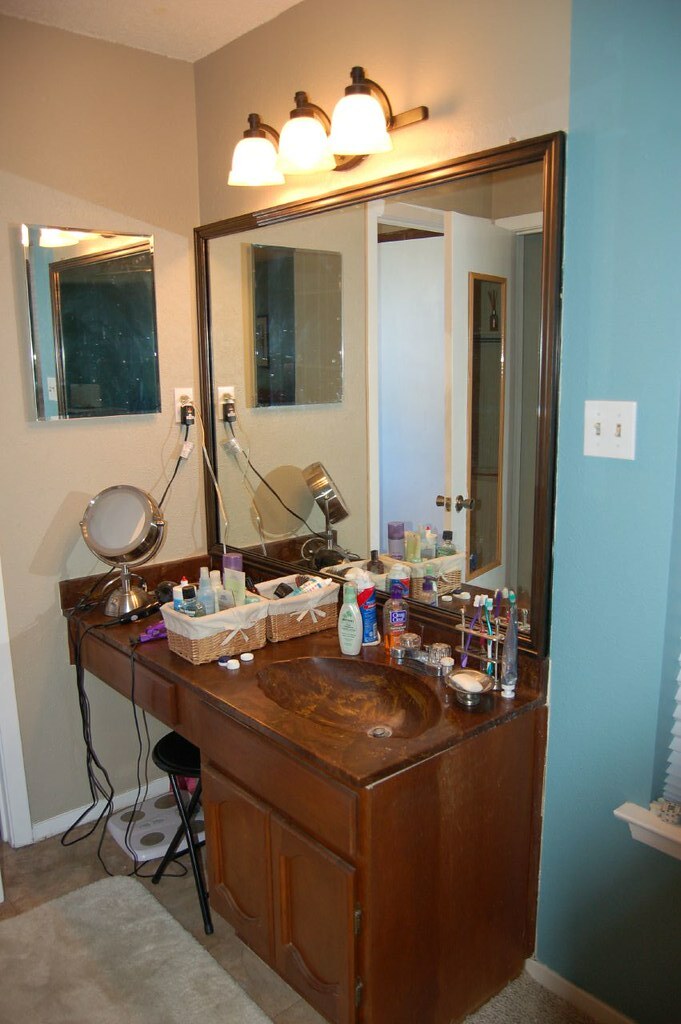The image depicts a sleek bathroom vanity set against a baby blue wall. The vanity, crafted from a dark material mimicking wood, features a rectangular design that is both long and narrow. At the right side of the vanity is a sink with a shiny silver drain and a short, elegant spigot with its handle positioned towards the back. The vanity is neatly organized with two baskets situated on the left side of the sink, containing assorted self-care items, tubes, and plastic bottles.

Adjacent to these baskets lies a metallic toothbrush holder, containing at least two or three toothbrushes, positioned close to the large mirror attached to the back of the vanity. In front of the toothbrush holder and nearer to the sink is a metallic soap dish. The vanity is arranged at an angle from the viewer’s perspective, reflecting part of a slightly open door to another room, the destination of which is unknown.

On the left wall, which is a plain tan color, hangs a smaller mirror with a metallic silver-gold frame. This smaller mirror, facing directly towards the viewer, has wires extending from it, indicating it is electrically powered and plugged into an outlet behind it. The large mirror on the vanity, however, is set at an angle and primarily faces towards the left of the viewer, capturing reflections off-image. The overall composition of the scene portrays a well-kept and thoughtfully designed bathroom space.